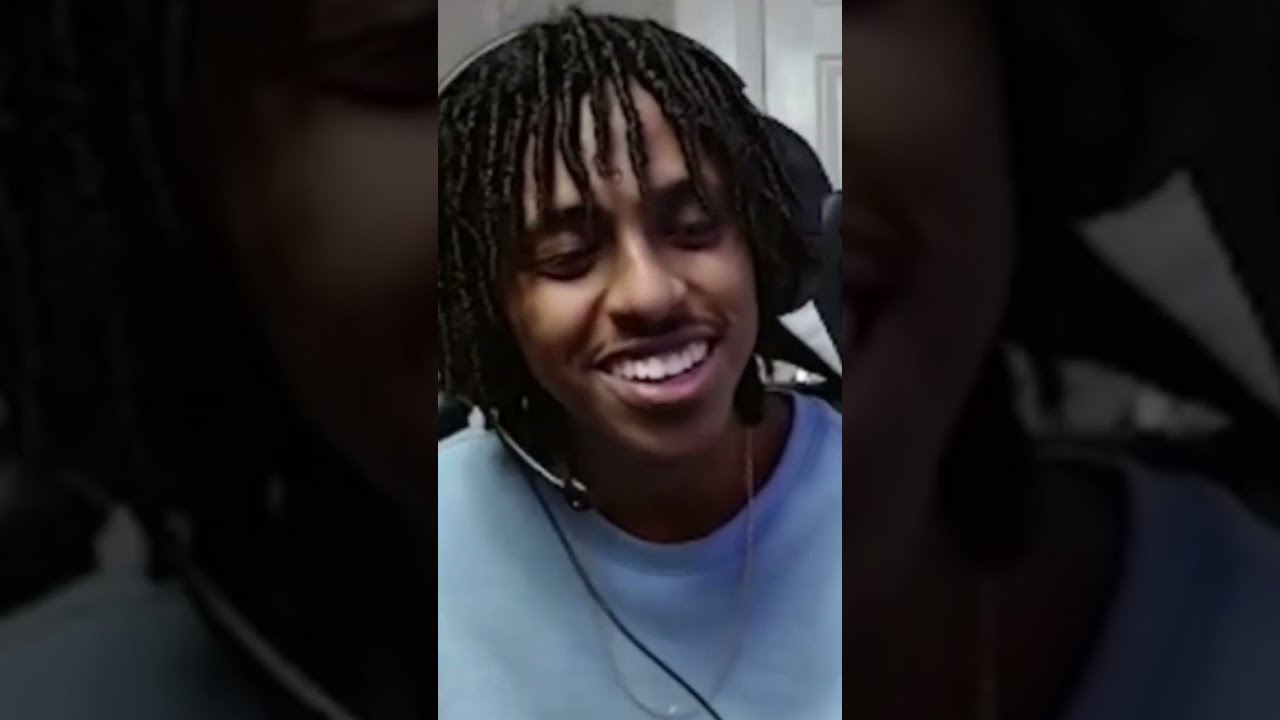This photograph is composed of three panels, with the central panel displaying the primary image clearly, while the two outer panels present heavily zoomed-in and underexposed versions of the left and right sides of the central image, both somewhat out of focus. The central image captures a cheerful young black man with long twists or braids in his hair and a neatly groomed mustache, suggesting a possible Jamaican heritage. He is wearing a light pastel blue or white shirt, accompanied by a gold chain around his neck. The man is engaged in a conversation, as evidenced by the gaming headset with an attached microphone that he is wearing. He is looking to the right, smiling brightly, and appears to be enjoying the interaction. In the background of the central image, there is a white door visible. The overall ambiance of the photo suggests that the man is content and enthusiastic, possibly engaging with an audience.